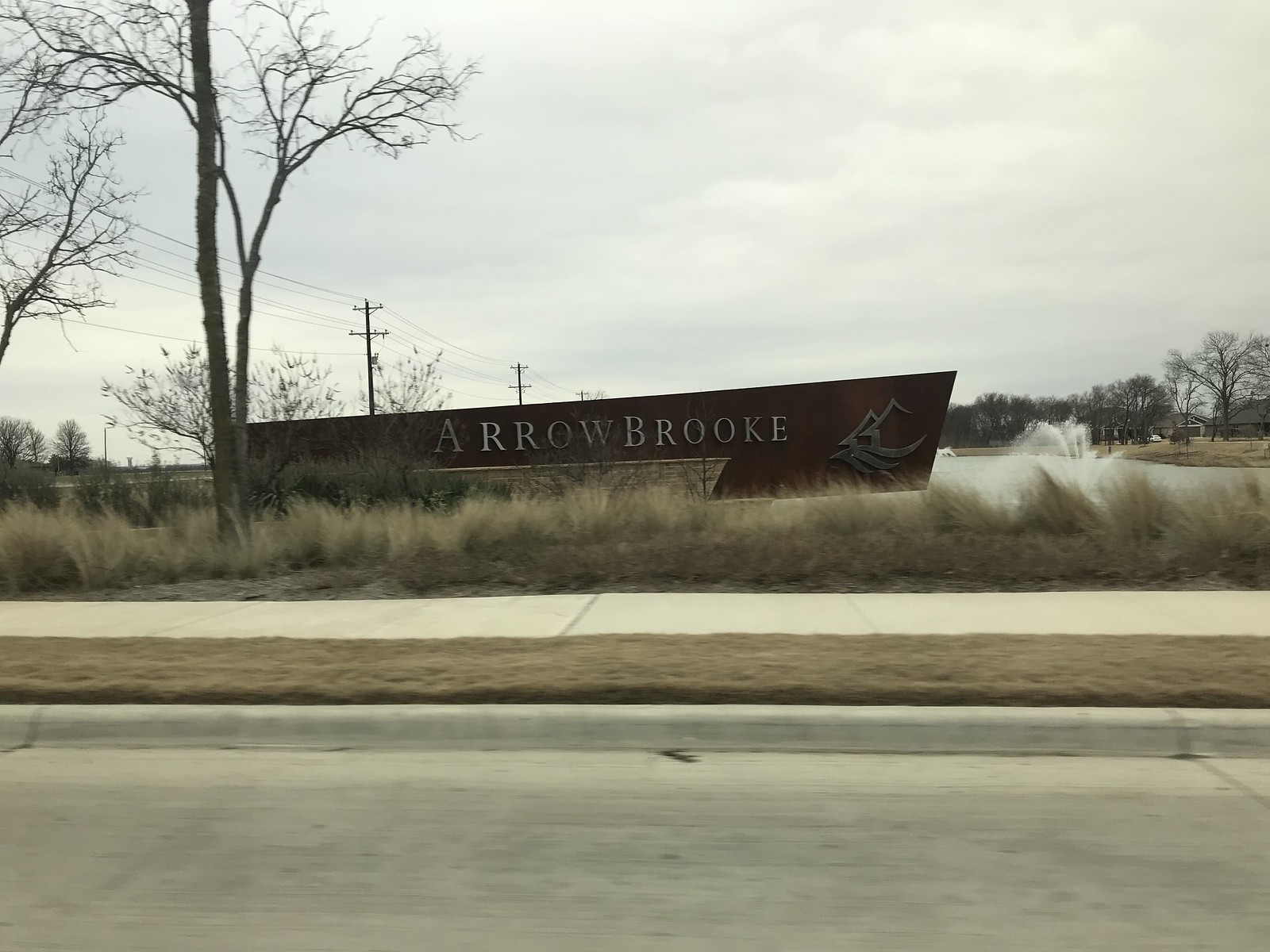This outdoor color photograph appears to have been taken from the perspective of a photographer standing on the side of a road. At the bottom edge of the image, a small section of asphalt pavement is visible, followed by a curb and a narrow strip of grass that has turned brown, suggesting the season is winter. Just beyond this, a sidewalk extends into the frame, bordered by more vegetation, primarily weeds.

Among the weeds stands a prominent sign. The sign is dark brown with silvery lettering that reads "Arrowbrook," likely indicating the name of a nearby facility, although the specific nature of the place is not provided. The overall scene is set against a backdrop of a gray, overcast sky filled with clouds, reinforcing the wintry atmosphere.

On the left side of the photograph, several leafless trees are visible, further emphasizing the seasonal context. Beyond the trees, in the distant background, a series of power lines can be seen stretching across the landscape, adding an industrial element to the otherwise natural setting.